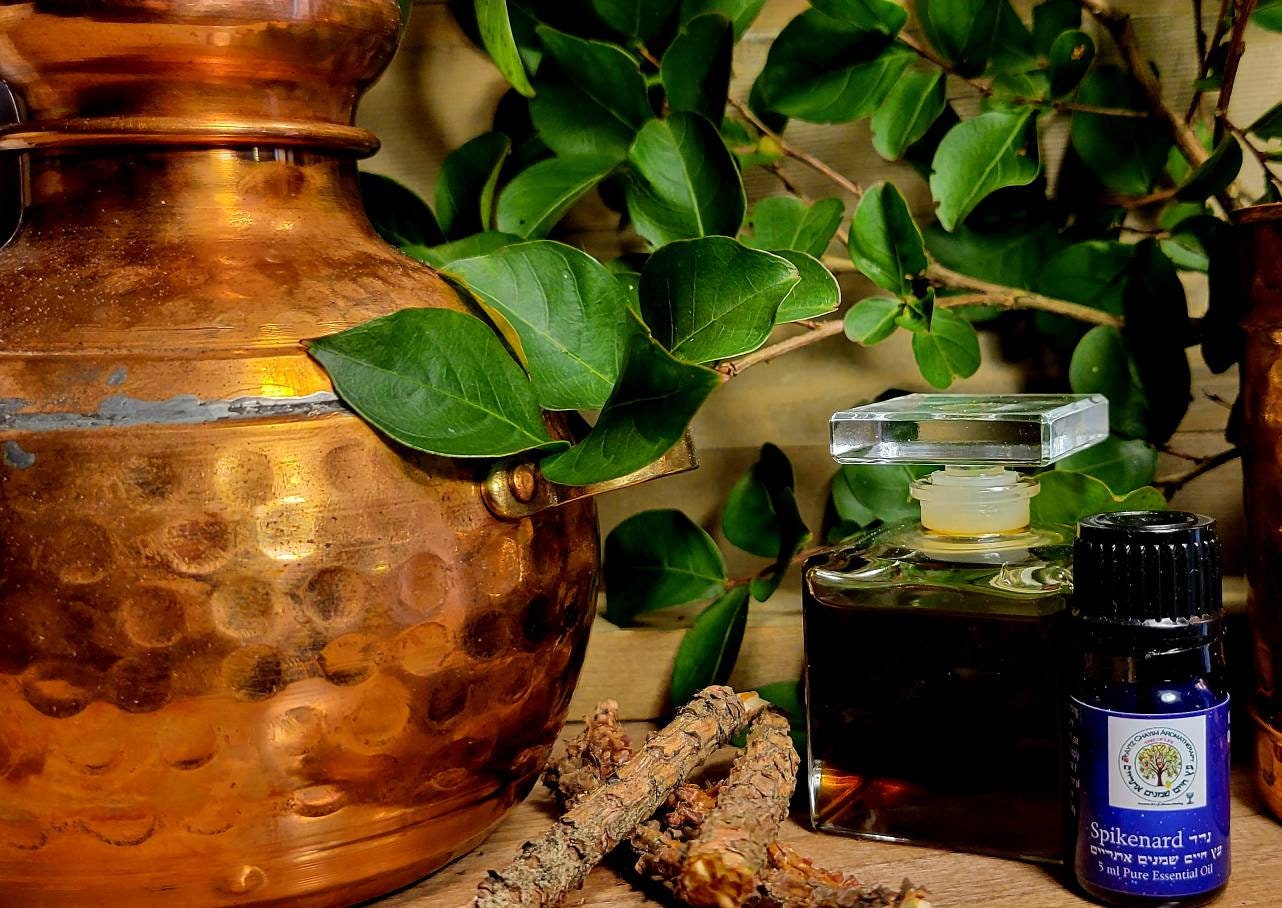In this captivating still life photograph, a prominent copper urn, featuring a textured, dimpled surface and a detachable top, commands attention on the left side of a wooden tabletop. The urn exhibits natural discoloration around its midsection, possibly from exposure to the elements, and boasts handles that might be brass or copper. Flanking the urn is a collection of vessels, including an amber bottle of essential oil with a dropper lid, and a perfume bottle filled with dark brown liquid, crowned by a crystal prism stopper. The scene is enriched by natural elements such as a luxuriant indoor tree with branches and green leaves, alongside pieces of bark, reinforcing the theme of traditional fragrances and natural aromas. The tabletop also hosts a can labeled "Spike Nerd Pure Essential Oil," completing this meticulously arranged tableau.